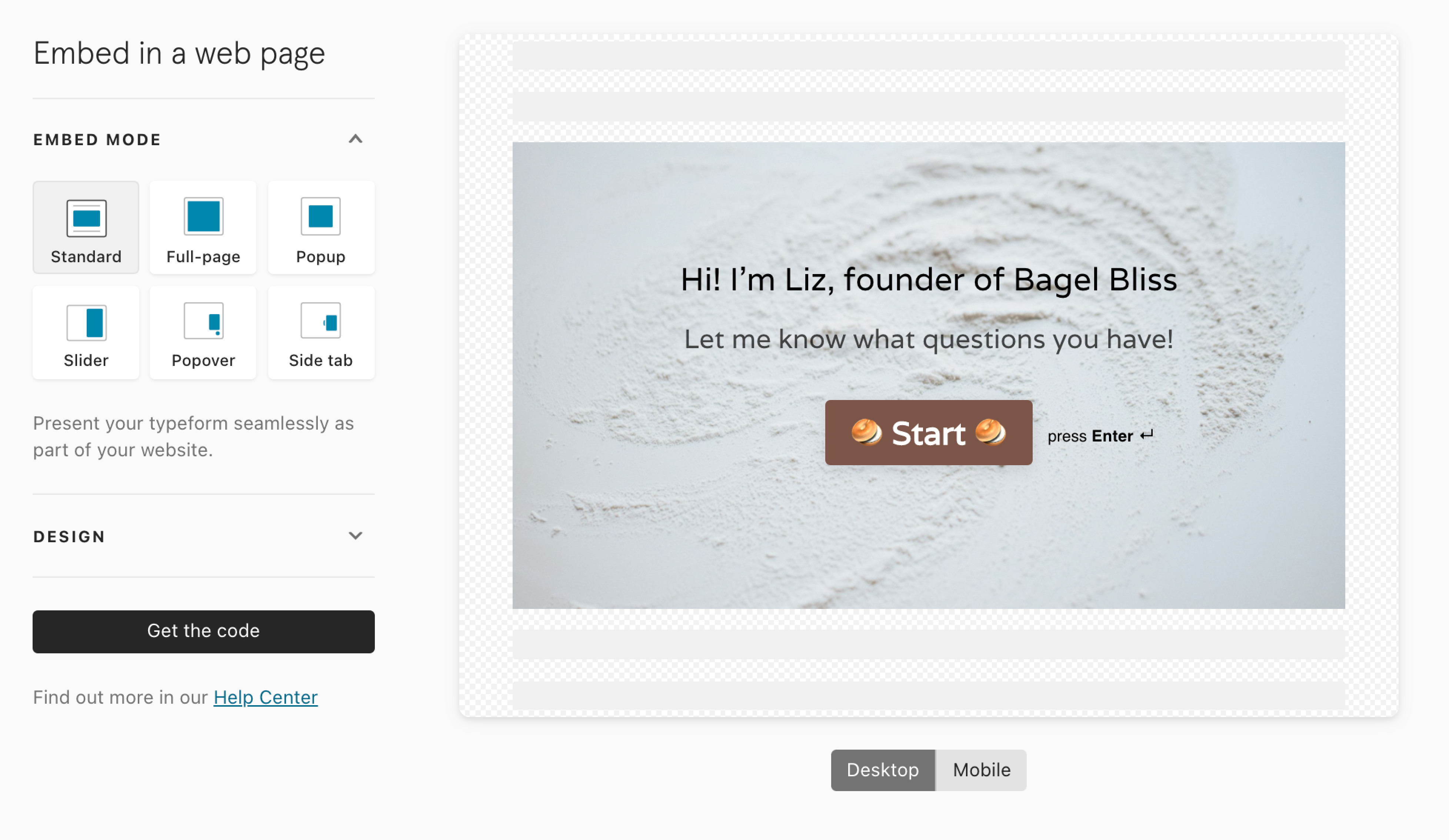The image displays a webpage interface focused on embedding options for a form. At the top, a section labeled "Embed in a Webpage" is clearly visible. Below this section, a row of embedding modes is presented, listed from left to right: Embed Mode, Standard, Full Page, Pop-Up, Slider, Pop-Over, and Side Tab. A sentence underneath these options reads, "Present your type form seamlessly as part of your website." An adjacent design element includes a downward arrow, indicating further clickable options.

A black box with white text that reads "Get the Code" is noticeable, suggesting it contains the embedding code. Additionally, there's a link to the "Help Center," highlighted in blue, inviting users to seek more information.

Within the selected "Standard" embed mode, there is a box featuring a conversational greeting from Liz, the founder of Bagel Bliss. The message states, "Hi, I'm Liz, founder of Bagel Bliss. Let me know what questions you have." Just below the greeting, a burnt orange box featuring two small bagels and the word "Start" in white text is visible, with the directive "Press Enter" nearby in black print.

Further down, the options "Desktop" and "Mobile" are specified, with "Desktop" currently selected, indicating the user's preferred working environment at the moment.